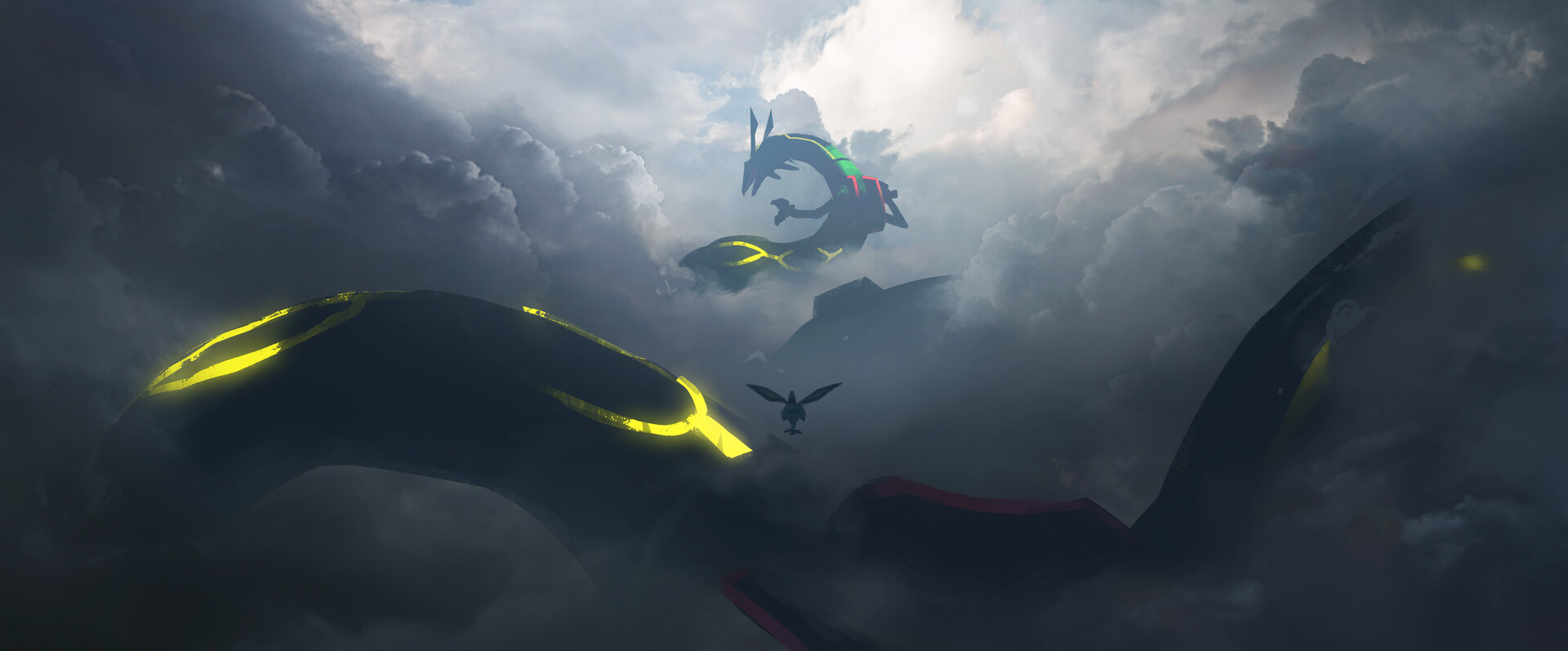In this mesmerizing digital illustration, a majestic dragon soars through a sky adorned with billowing clouds. The dragon's serpentine body, silhouetted against a stark backdrop, stretches across the image, creating a sense of depth and perspective. The dragon's head is small and positioned at the center, where it is bathed in the brightest light, giving it a mystical glow.

Its elongated, snake-like form is accentuated by a pair of prominent fangs and distinctive yellow markings that emit a soft, ethereal glow. The dragon's head is crowned with two sets of horns—two arcing gracefully above and two jutting below. Further along its body, near its small, defined arms, there are green and red markings that provide a splash of color against the silhouette.

In the near-center of the image, just in front of the dragon, there is an intriguing, three-pointed object with radiating lines and a stand-like base. Its mysterious presence adds an enigmatic element to the scene, leaving viewers to ponder its significance.

Surrounding the dragon, the clouds twist and churn, with the brightest light emanating from the center, gradually fading into darker, stormier edges. This contrast in illumination adds a dramatic tension, highlighting the dragon's dominance in its celestial domain.